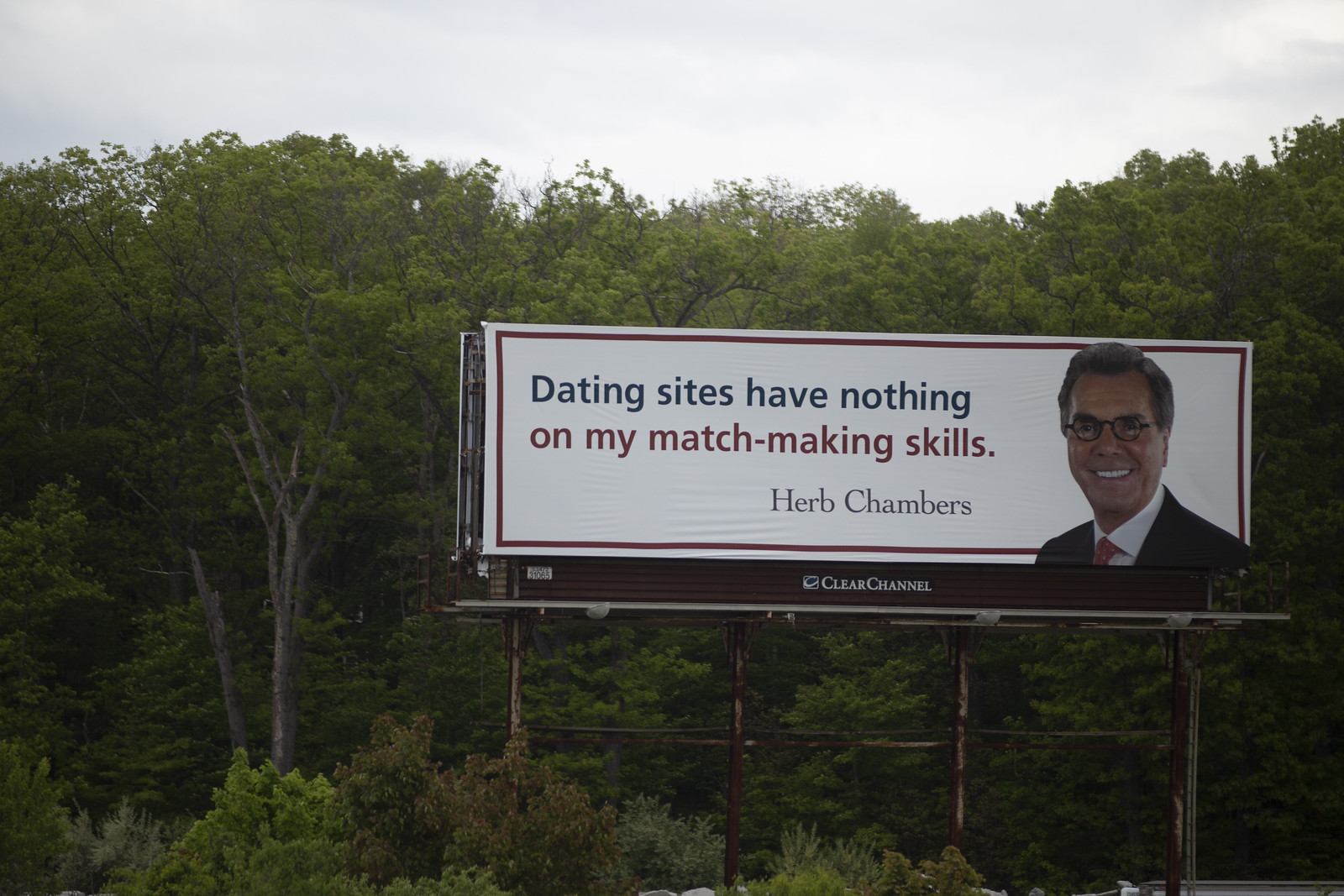This real-life photograph captures a prominent billboard advertisement prominently featuring a white backdrop with bold text. The blue text across the top reads, “Dating sites have nothing,” followed by red text underneath stating, “On my matchmaking skills.” Centrally placed below this text is the name “Herb Chambers” in title case serif letters. To the right side of the billboard is a lifelike portrait of a man, identified as a white man with gray hair and black glasses, who is smiling. He is dressed in a black suit paired with a white and red tie. The advertisement is enclosed within a red border.

Supporting the billboard are four posts, which appear aged and rusty, anchored into the structure amidst a backdrop of dense, tree-filled scenery. The treetop landscape spans the majority of the background, creating a lush and wooded visual setting. Above the trees, occupying roughly the top 10% of the image, is an overcast sky that casts a pallid daytime light with predominantly gray and white clouds, hinting at a dreary day. Additionally, at the base of the billboard structure, there is a logo reading “Clear Channel,” indicating the company that owns the billboard.